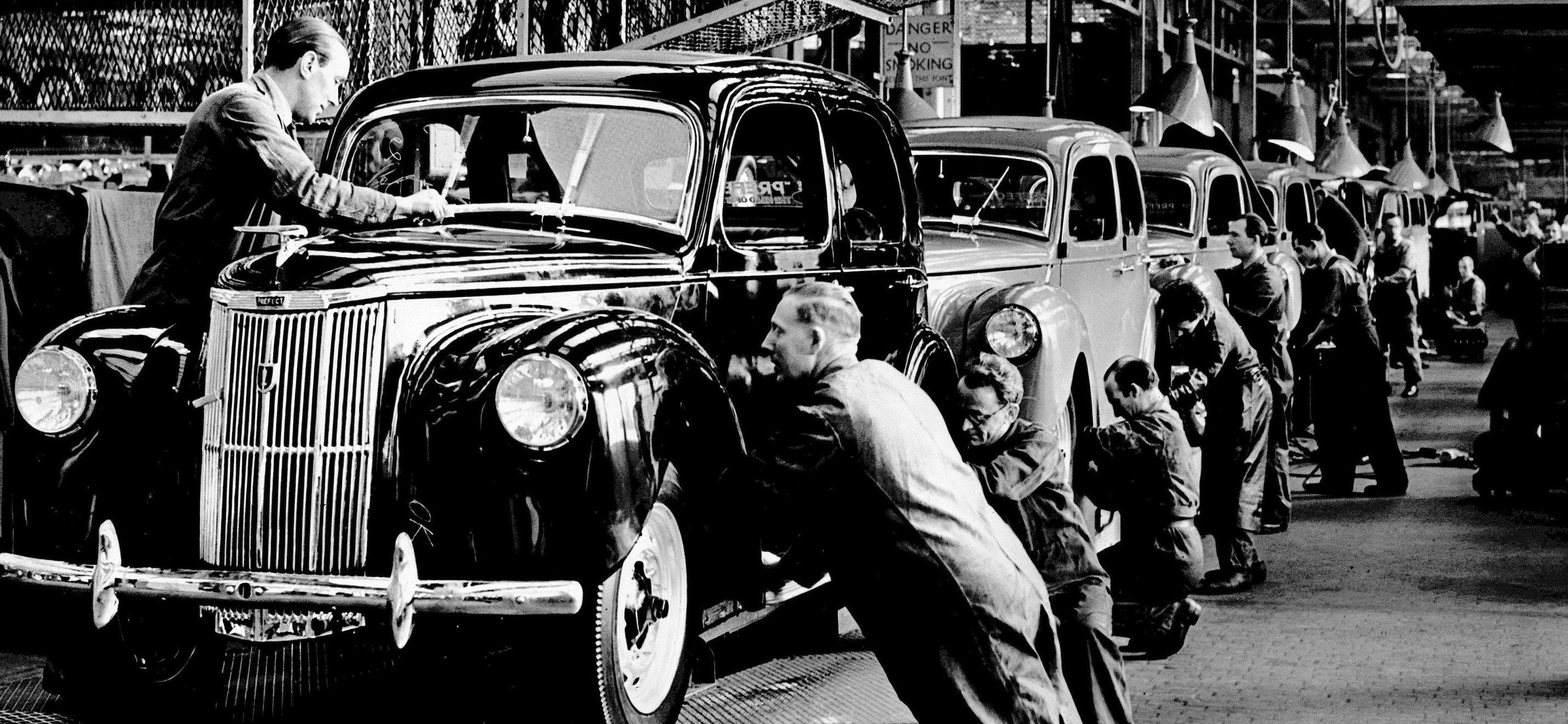This detailed, black-and-white vintage photograph from the 1920s to 1940s captures the bustling scene of an industrial car factory assembly line. A row of men, mostly dressed in work clothes and overalls, diligently attends to various tasks on the old model cars. On one side, eight men can be seen, with another man, distinguishable in a suit, inspecting the windshield wipers. The assembly line stretches from the left-hand corner to the right-hand corner, showcasing several similar-looking cars, one prominently polished black, followed by mostly white cars. The environment is filled with industrial elements such as hanging lights, metal grates, and cautionary signs like "danger" and "no smoking." The workers, engrossed in their meticulous roles, use tools to screw in parts and add pieces to the vehicles, all contributing to the creation of these vintage automobiles.